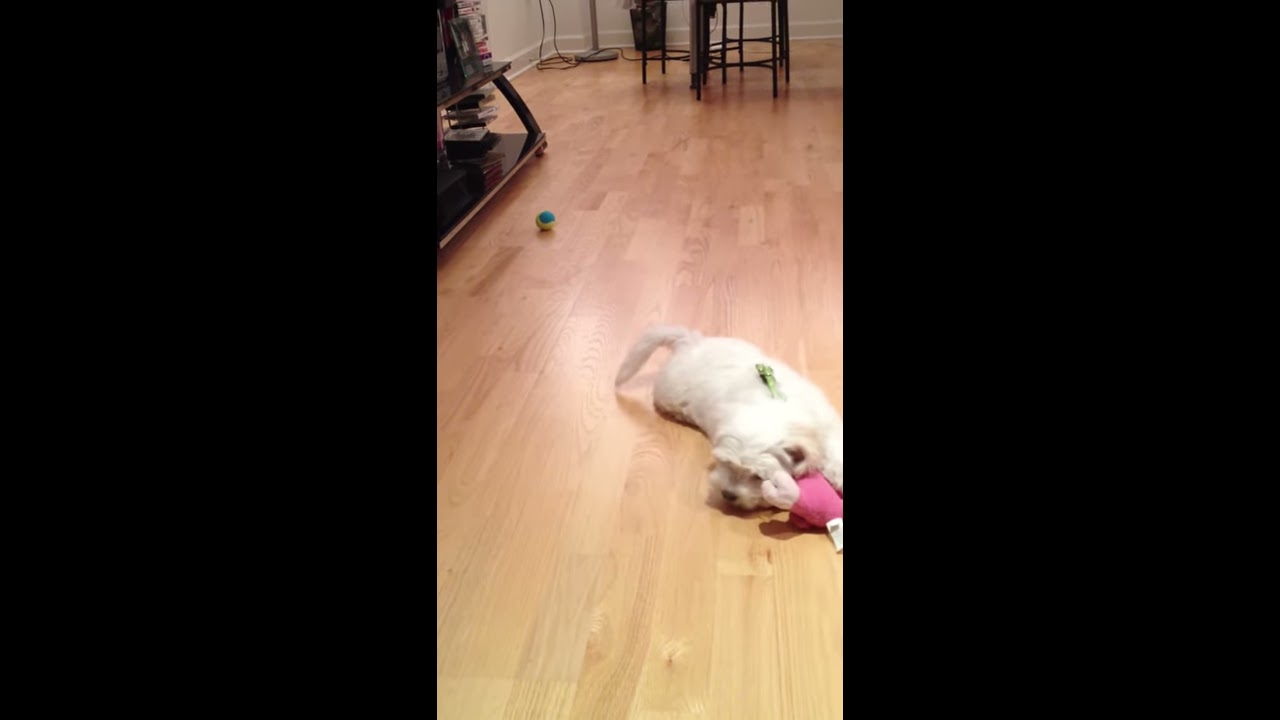The photograph captures a cozy living room scene inside a home, presenting a small, white dog lying on light brown hardwood flooring. The fluffy dog, with distinctive eyebrows, appears to be in the middle of playing next to a pink toy. Although the dog’s playful posture initially made it challenging to discern its species, it is clearly a dog. Also visible in the foreground is a second toy, a small green one that rests on the dog's body. The background of the image is detailed with various elements: a yellow and teal tennis ball, a black treadmill, and some chairs which seem associated with a table. The backdrop also features the bottom part of an entertainment system with two shelves, a white wall, and the base of a floor lamp situated next to the table or chairs. This picture, occupying the center panel of three, stands out against the black left and right panels, and it appears text-free.